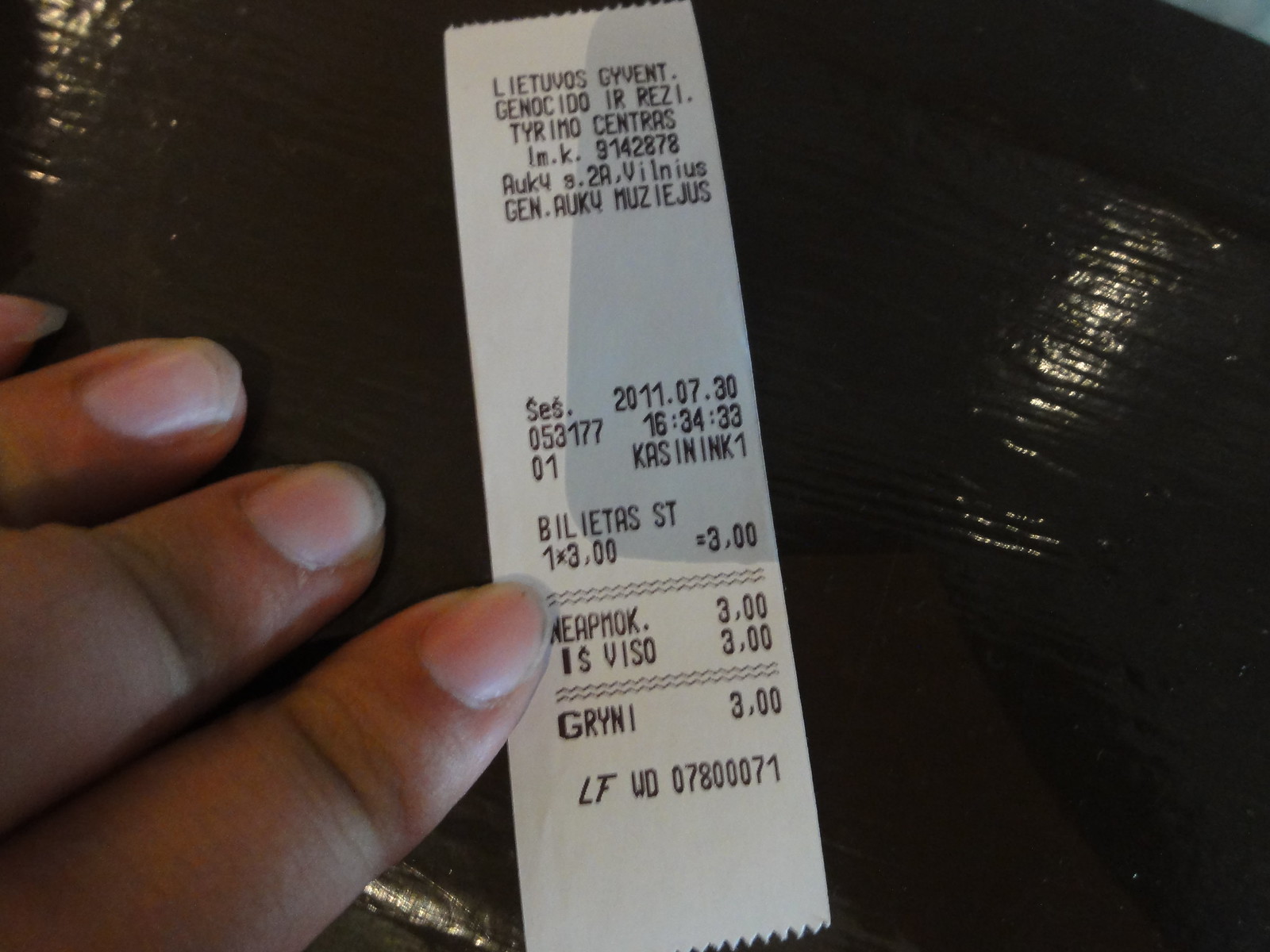The image features a square-shaped photograph with a receipt positioned prominently in the center. The receipt is rectangular with a white background and black text. To the left of the image, there are four visible fingers, with the index finger directly touching the receipt. 

The text on the receipt displays from the top:
- "LIETUVOS GYVENT"
- "GENOCIDO IR REZI"

Additional details in the text are partially visible, hinting at more content below. The picture is clearly focused on highlighting the receipt and the interaction with it, providing a close-up view of the text.